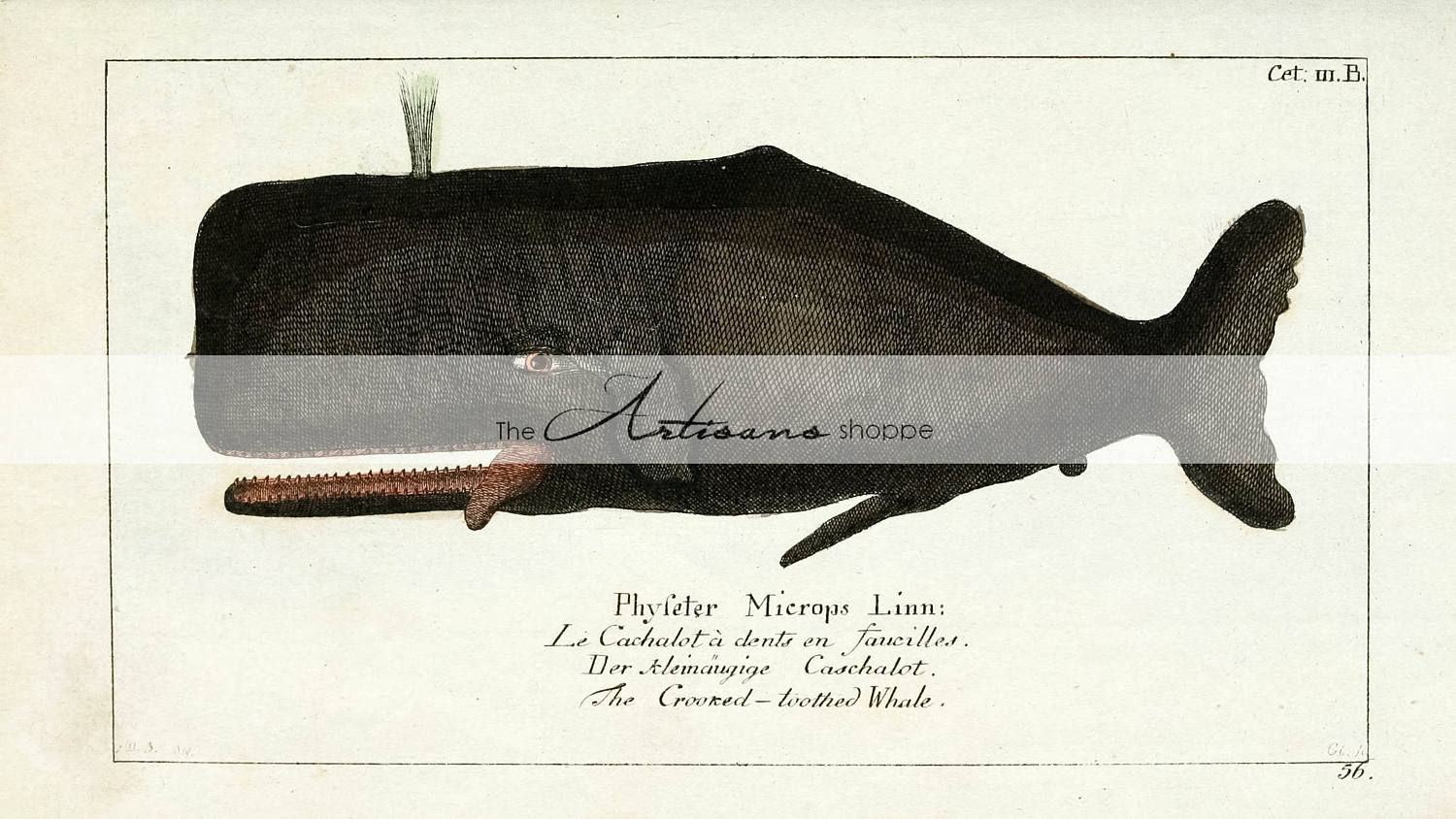The image is a stylized drawing of a black whale prominently displayed on a white background with a thin black rectangular border. The whale, labeled as the "Crooked Tooth Whale," is depicted with a red mouth and numerous teeth, oriented from right to left—tail on the right, head on the left, which is rectangular in shape. The whale is also spouting water from its blowhole. Overlaying the whale is the text "The Artisan Shop." Below the drawing, the text reads "Pfeifferter Microps Linn" and includes a multilingual caption with phrases like "le cache à l'eau" and other complex words that appear to be in French and German. In the top right corner of the image, there are letters reading "CET M.B" and in the bottom right corner, the number "56" is visible. The drawing is set on a brown piece of paper, adding an artistic, vintage feel to the overall presentation.